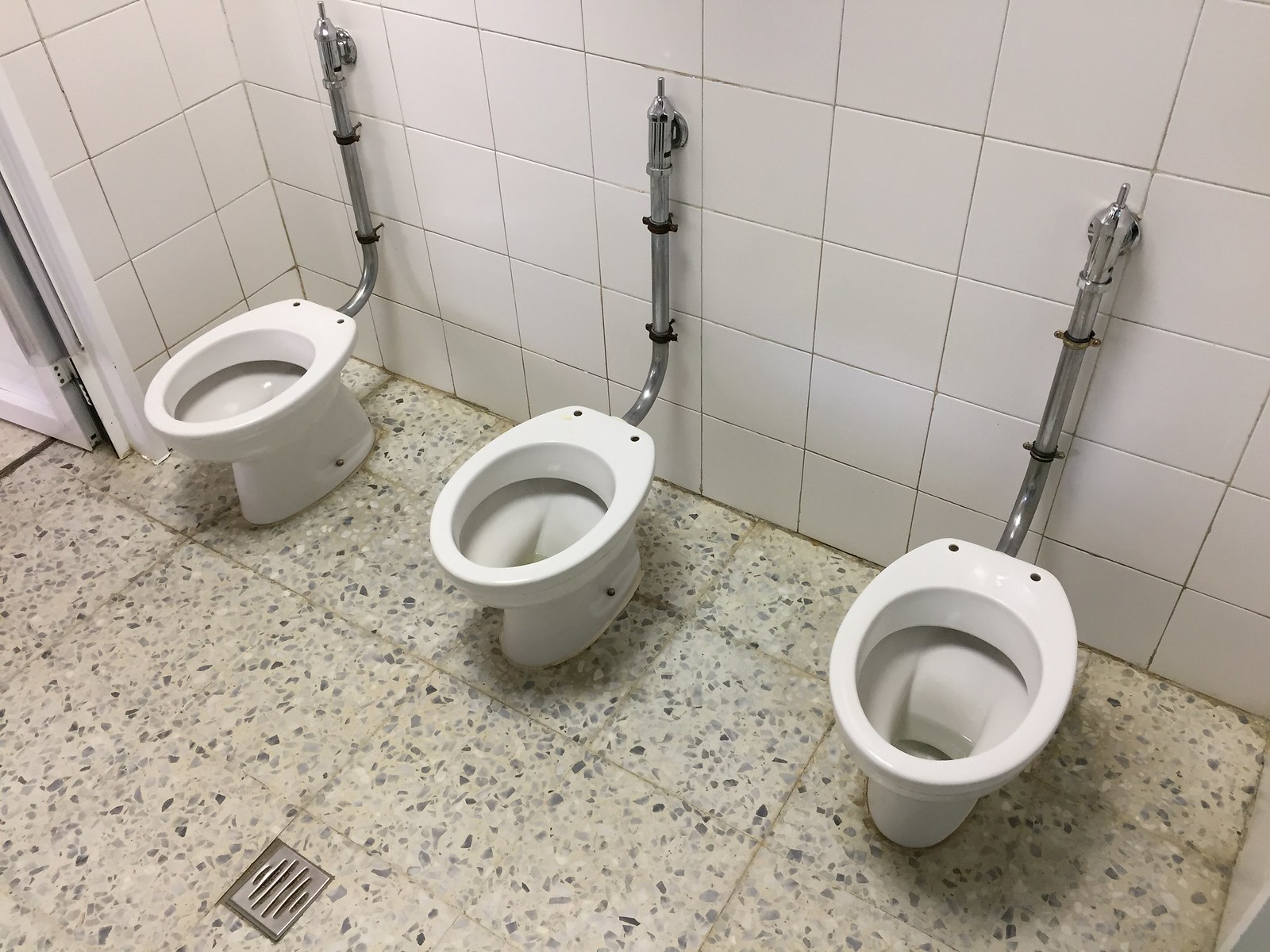The image shows the interior of a men's public restroom featuring three white porcelain urinals mounted against a wall. Each urinal is equipped with a silver pipe running up to the wall for plumbing, ending in a long cylindrical flush button. The urinals are deep but unusually low, and they lack dividers between them, making it a very open and public setup. The walls are covered in white tiles, and the floor is a yellowish-white color with black and gray specks, resembling a marble design. A small silver drain is situated in the center of the floor. The overall view is angled, providing a clear perspective of the space and the urinals.